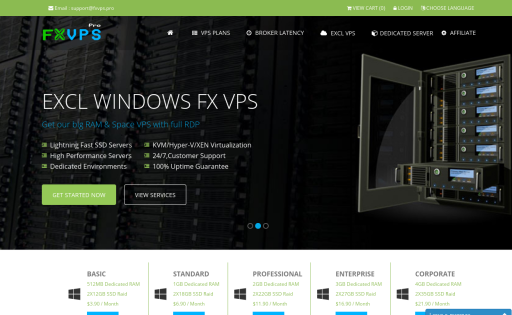In the image, the top section of the webpage features a green header with blurry tabs. On the top left, the text reads "Email support at fxvps.pro". On the top right, it says "You can't log in" and "Choose language," all against the green background. Below the header, the background displays a server rack with server machines.

The main content starts on the top left with the company logo "fxvpspro": "fx" is in green, "vps" is in blue, and "pro" is in white. White text tabs at the top display navigational options: Home, VPS Plans, Broker Latency, Exclusive VPS, Dedicated Server, and Affiliate.

In the center-left of the main page, promotional text reads "Exclusive Windows FXVPS - Get our big RAM and space VPS with full RDP" in blue, with specifications listed in white. Each specification is accompanied by a green square:
- Lightning Fast SSD Servers
- High-Performance Servers
- Dedicated Environment
- KVM, Hyper-V, Xen Virtualization
- 24/7 Customer Support
- 100% Uptime Guaranteed

Two buttons are positioned on the bottom left: "Get Started Now" in green, and "View Servers" in black.

On the right side, an image of a grey server box with blue and yellow LEDs is shown. At the bottom, various plan options are listed: Basic Plan, Standard Plan, Professional Plan, Enterprise, and Corporate, with the plan descriptions in green, though they are not readable.